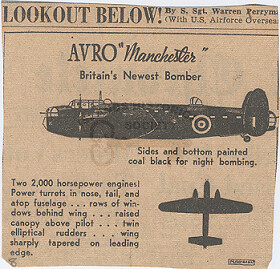The image depicts a vintage newspaper or magazine article, possibly from the 1930s or 1940s, printed on a gray or tannish background. At the very top, a bold headline in black letters reads "Look Out Below!" followed by a subheading "by South Sergeant Warren Perryman (U.S. Air Force)" in parentheses. Underneath this, a horizontal black line encases the main content.

Central to the article is a large black airplane featuring a prominent white bullseye symbol on its side, along with white dotted lines. Above the plane, the text proclaims "AVRO Manchester: Britain's Newest Bomber." Below it, another image shows the top view of the black plane, with the caption "Side and bottoms painted coal black for night bombing."

To the left of this bottom plane image, descriptive text in black provides technical details: "Two 2,000 horsepower engines power turrets and nose tail and up top fuselage. Rows of windows behind wings. Raised canopy above pilot. Twin elliptical rudders. Wing sharply tapered on the leading edge." Additionally, an '8' in black and some unreadable symbols or text appear at the bottom right corner. The overall tone and the paper’s aged look, suggested by its color and print style, imply that this article is likely from an old publication.